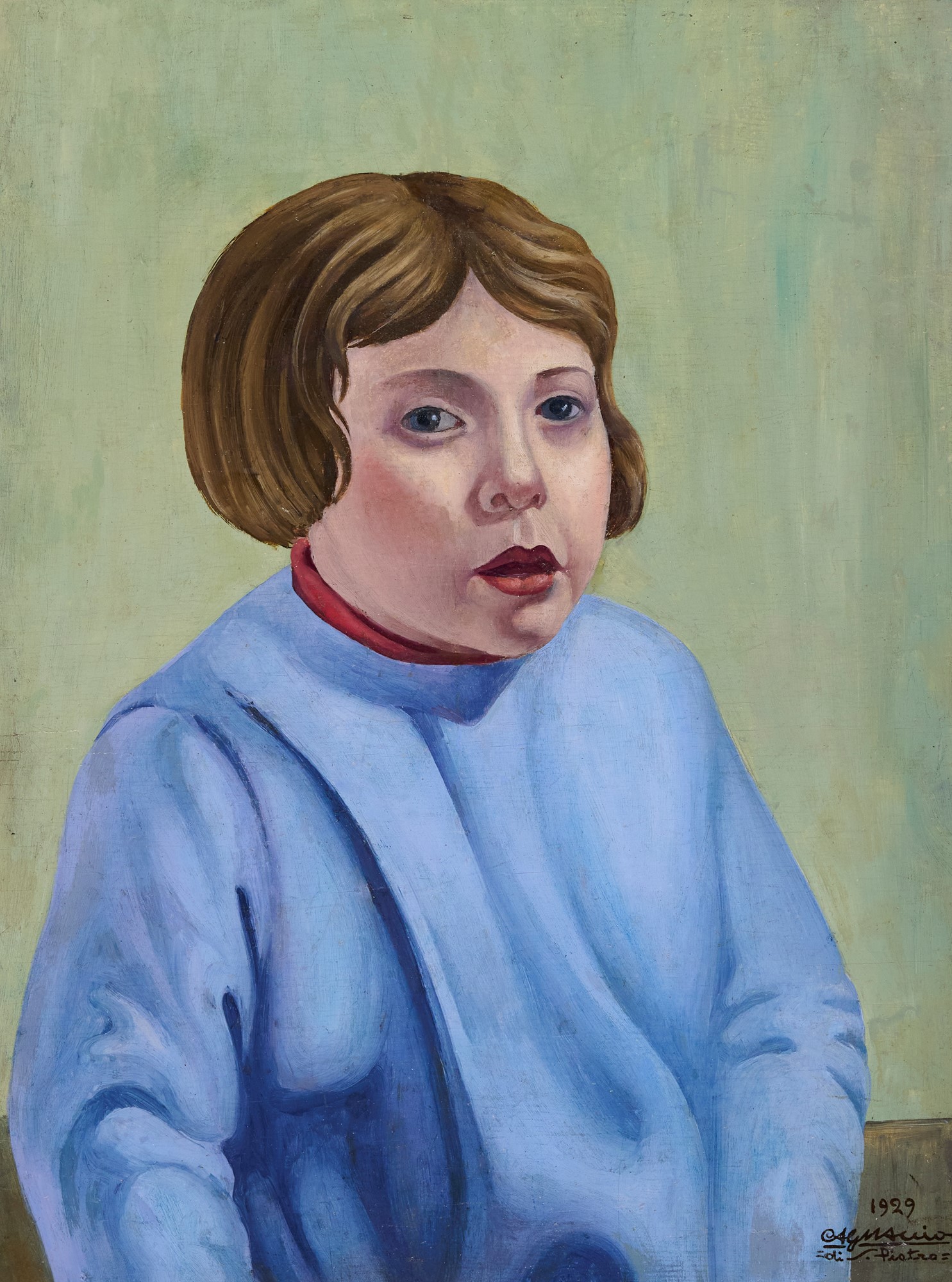This is a detailed painting of a feminine-looking figure, possibly a woman or a young girl, depicted against a pale greenish-gray background. The figure, with short brown hair that reaches mid-cheek, has distinguishable features including round, slightly bluish-tinted skin, luminous blue eyes, and full, bright red lips that are slightly parted, revealing a hint of the lower teeth and a dark interior of the mouth. She is dressed in a loose-fitting, sky blue sweatshirt, and a red collar from the shirt underneath peeks out. The floor visible on either side of her body is a grayish color. There is a signed indication at the bottom right, with the date "1929" inscribed in black numbers above the signature. A notable detail is the name “Agnes Hughes” along with the unclear initials “PTRO” beneath it.